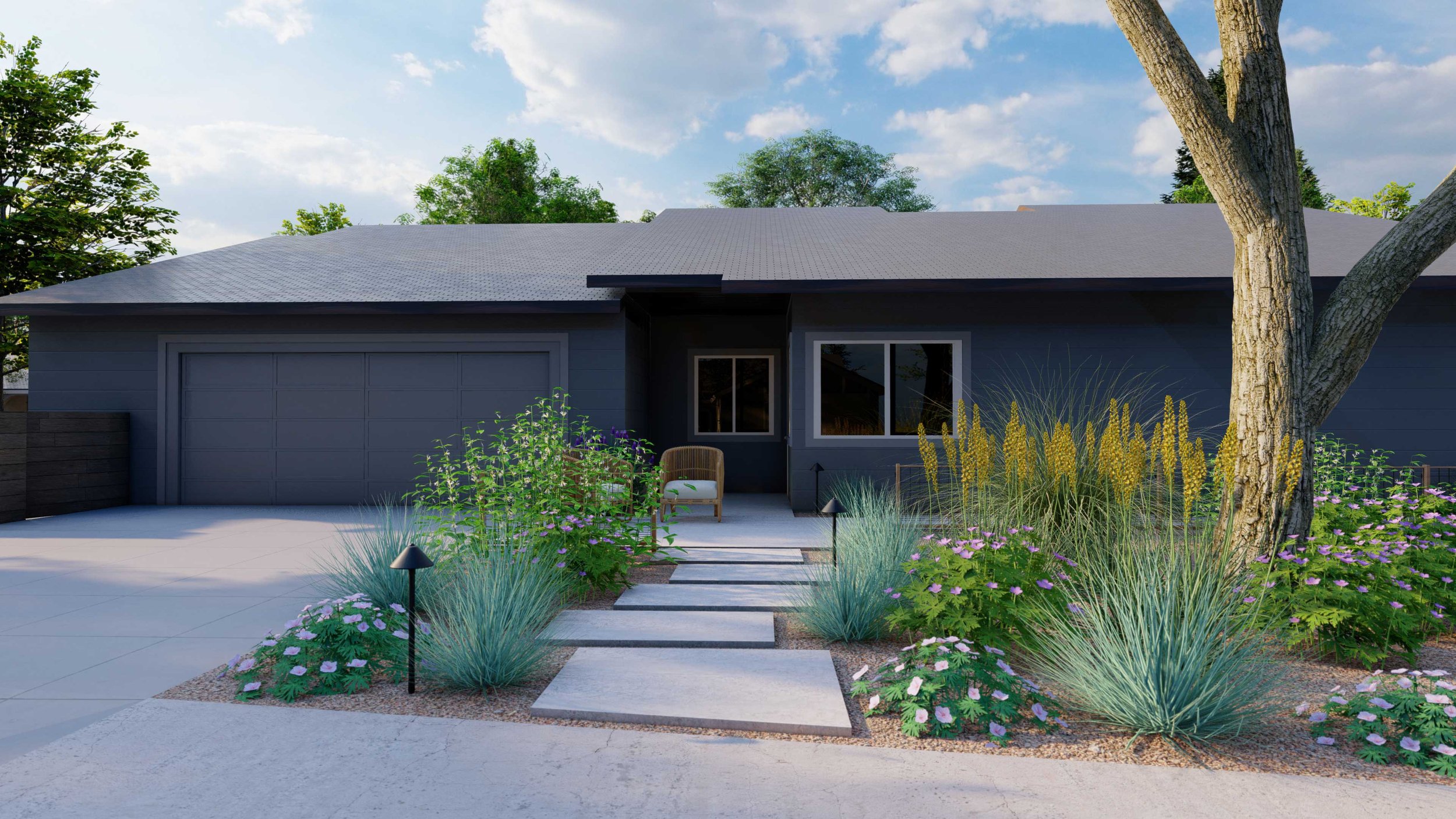This color photograph captures the picturesque front view of a ranch-style, single-story house, likely situated in the southwestern United States. The house is painted gray and features a matching gray roof, complemented by a two-car garage with a single long gray door. The house is accented by two prominent windows, both with white frames—a window recessed into the entryway and another on the front facade.

Leading to the front entrance is a sidewalk of large, offset paving stones. The walkway is flanked by various grasses, decorative plants, and flowers, including some purple and pink blooms. At the end of the walkway, there are two brown lawn chairs with clean, white upholstery positioned invitingly. An additional wicker chair with a big white cushion is nestled in the recessed area by the front window, adding to the cozy, welcoming atmosphere.

The yard replaces a traditional lawn with sand and pebbles, highlighting the region's characteristic landscaping. Despite the arid soil, the garden is lively with multiple green plants and the trunk of a sizable tree in the foreground. Although the leaves of the tree are not visible, branches stretch towards a bright blue sky scattered with a few white clouds, creating a serene backdrop. The tops of other trees and more green foliage can be seen in the distance, contributing to the tranquil setting.